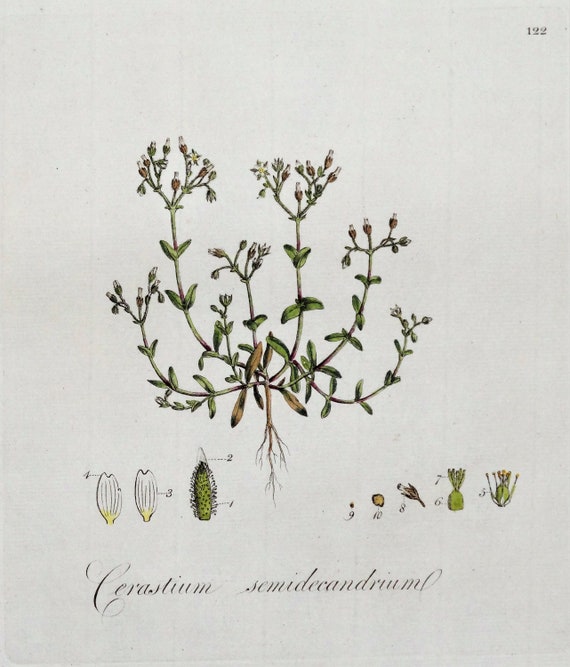This detailed scientific illustration depicts a small plant named Cerastium semidecandrium, presented on an off-white background that evokes an old-fashioned botanical drawing. The plant features multiple branches with oblong leaves in shades of green and brown. At the end of each branch, forking structures bear clusters of compact white flowers with yellow bases. Below the main illustration, a series of detailed drawings depict the blooming stages of the flowers, from the unopened pods to the mature blooms. On the opposite side, additional diagrams show the development of the seeds and seed pods, with each small illustration meticulously labeled. At the bottom of the page, the plant's scientific name, "Cerastium semidecandrium," is elegantly written in a dark, cursive script.